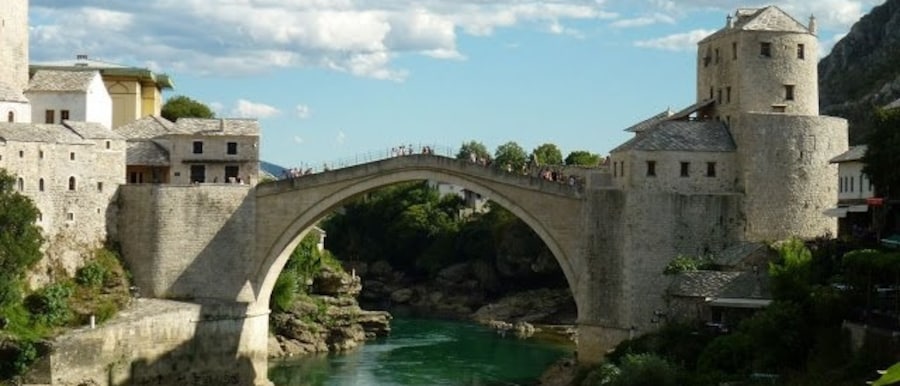This vibrant daytime photograph captures a picturesque medieval scene dominated by a historic stone and concrete bridge that arches gracefully over a green-tinted river. The bridge appears to be a popular spot, dotted with people crossing between two distinct areas. On the left, the riverbanks host quaint, stone-built village houses, creating a charming contrast with the more imposing, castle-like structures on the right, which seem to cling to the side of a cliff or mountain. Above, the vibrant blue sky is adorned with a few fluffy white clouds, while lush green trees frame the background and the edges of the image. The sunlight bathes the scene in a bright, clear light, enhancing the vivid colors and fine details of this captivating landscape, making it appear almost like a historical landmark or a tourist attraction.